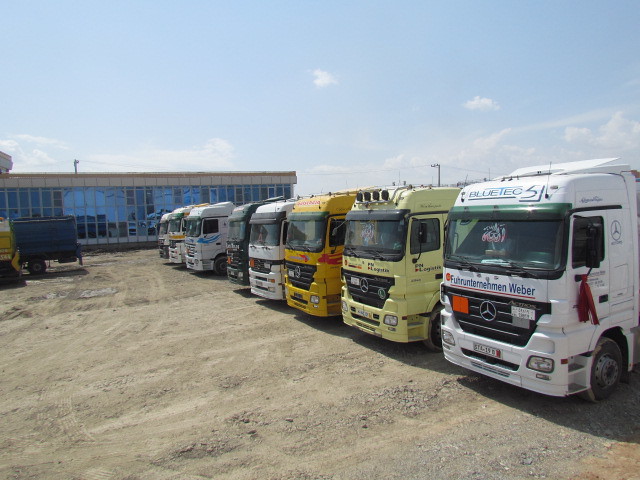This image captures a work yard in a foreign country, characterized by a line of eight semi-trucks parked on a light gray gravel surface. The trucks, primarily Mercedes-Benz, are organized from right to left in the following colors: white, light yellow, bright yellow, white, black, white, and possibly black or white trucks at the far ends. Distinctive details such as "Blue Tech," with the number 5 and the name "Weber," are visible alongside the Mercedes logo on the first truck. In the background, a building with many blue-tinted windows can be seen, along with telephone poles and wires crisscrossing overhead. Additionally, a blue dump truck is visible in the distance to the left. The scene is set under a light blue sky with a few small clouds, adding to the overall tranquil yet industrious atmosphere of the yard.